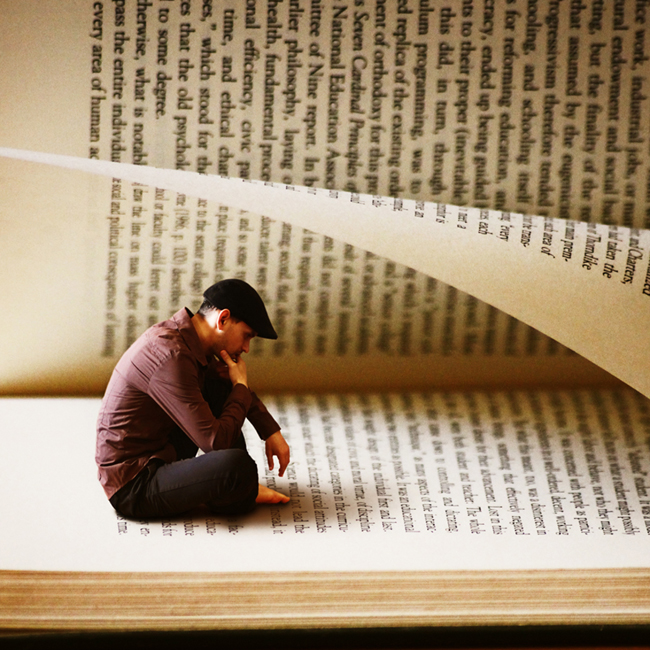The image portrays a fascinating scene of a man in deep contemplation, captured in a seemingly miniature form as he sits on the page of an enormous open book. The book is positioned flat with its back laying down, offering a side view of the intersecting pages. One of these pages is only halfway open and sloping down like a gentle wave. The man, positioned at the bottom left corner of the partially turned page, is dressed in a black newsboy cap, a reddish-purple long-sleeve button-up shirt that covers his arms, and black pants. He sits cross-legged, barefoot, and with an introspective posture—his left hand under his chin and his right arm hanging down towards his feet. His gaze is fixed upon the lines of text beneath him, seemingly lost in thought. Below him, layers of unopened pages and a dark trim under the book cover provide a subtle backdrop, emphasizing the surreal nature of this strikingly imaginative photograph.